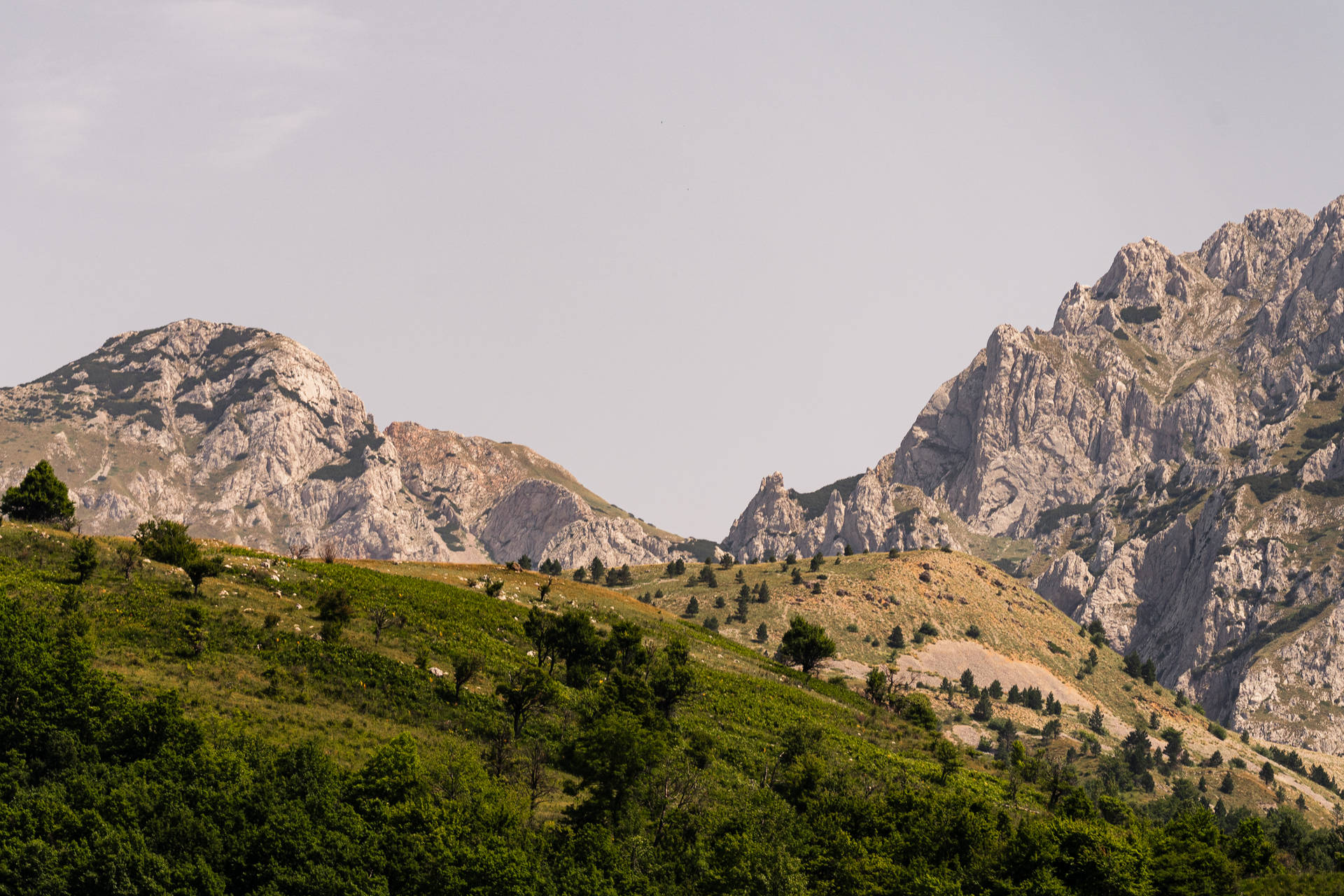This vertical rectangular image captures an enchanting landscape dominated by a rugged mountainous range. The backdrop showcases a blue sky partially shrouded by hazy gray and white clouds, especially concentrated on the left. The mountain range stretches continuously from left to right, with jagged, grayish-tan rocky peaks that are more prominent and towering on the right side. Among these peaks, hints of white suggest either lighter rock surfaces or lingering patches of snow.

Descending from these rocky elevations are verdant, sloping hills punctuated by patches of green grass and scattered trees. The right side of the green hills noticeably slopes downward, adding a dynamic layered effect to the scene. These lower hills appear more lush and verdant with dense, dark green grass and trees as they approach the viewer, creating a sense of depth in the foreground.

The foreground further features a grassy hill with earthy tones and clusters of greenery including bushes and trees with brown stems and branches. The bottom edge of the image reveals a smaller, vividly green hill adorned with a dense row of dark green trees, contributing to the lushness of the scene. There are even some indications of animals, perhaps sheep, dotting the greener areas, enhancing the pastoral charm of this captivating outdoor day scene.